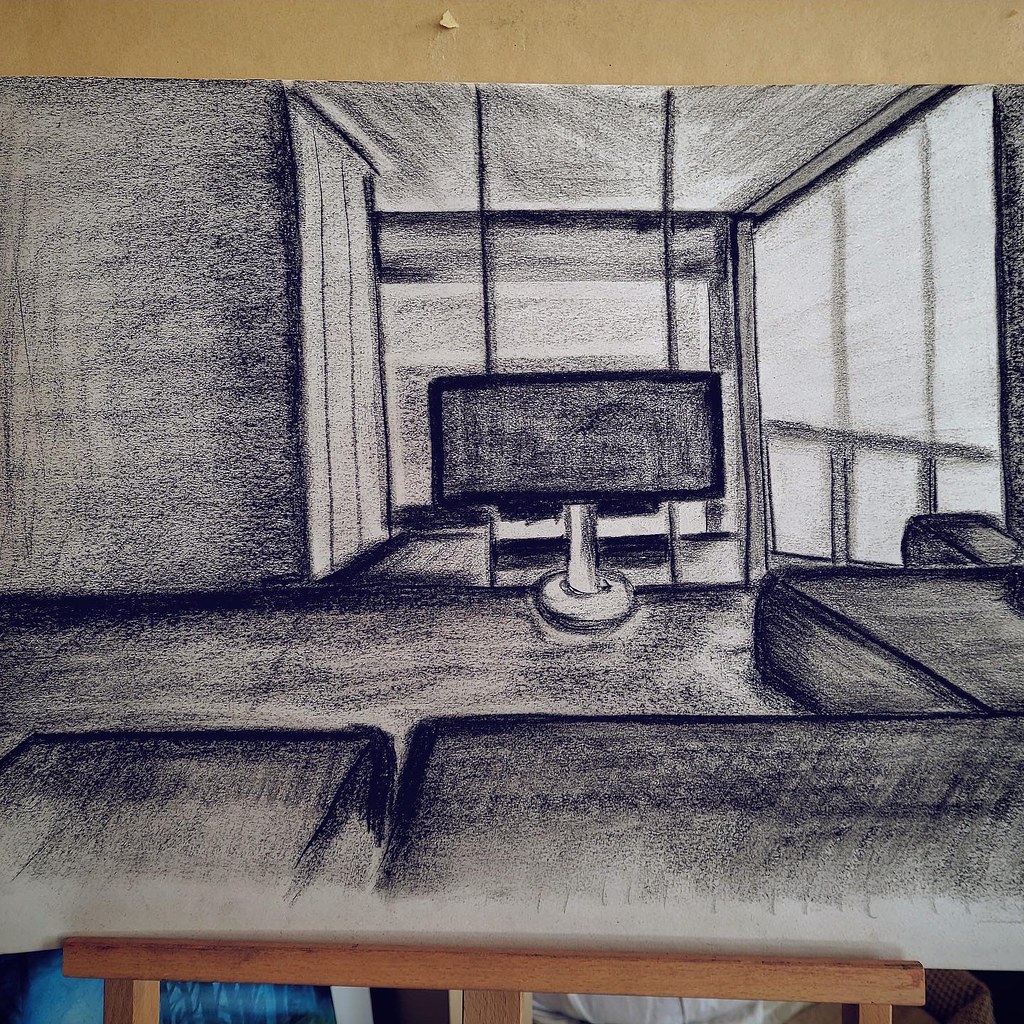A meticulously detailed black and white pastel drawing captures the perspective of a person reclining on a couch, intently watching a large television or monitor. The artist's masterful shading creates a striking play of light and shadow, with a shade partially drawn over the windows, through which you can see the contours of the dividers and the subtle reflection of ambient light on the opposite wall. As the eye moves deeper into the composition, the atmosphere grows progressively darker, enhancing the depth and realism. The screen of the TV or monitor appears almost pitch-black, while the surrounding ceiling is enveloped in shadow, yet every element remains distinctly recognizable due to the nuanced gradations of black, grey, and white. The artwork itself appears to be displayed either at the back of a chair or the foot of a bed, suggested by a visible rail or possibly an easel running along the bottom edge of the image. This thoughtful presentation further adds to the drawing's immersive and introspective quality.